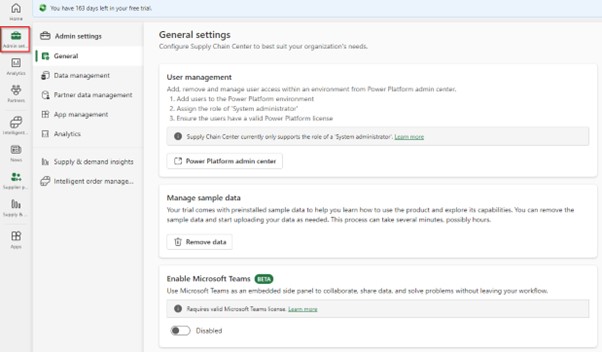This image is a partially cut-off screenshot of a free trial for an unspecified program. In the top-left corner, there is a home icon accompanied by the word "Home." Below this, there are eight additional icons with illegible text beneath each. 

To the right of these icons, there is a vertical menu. The first item is "Admin Settings," which is indicated by a briefcase icon. Below that, a highlighted link labeled "General" features an icon of a square containing a circle. The subsequent links are titled "Data Management," "Further Data Management," "App Management," "Analytics," "Supply and Demand Insights," and "Intelligent Order Management." Each of these links presumably navigates to different sections within the same page.

The main portion of the page is dedicated to General Settings, with the heading "Configure supply chain center to best suit your organization’s needs." Below this, there is a sub-header "User Management" with some accompanying text. Users can select options such as "Manage Sample Data," "Remove Data," and the option to "Enable Microsoft Teams," which is marked with a "Beta" tag indicating it is in testing. There is also an option to disable this feature.

The overall color scheme consists of a very light gray or off-white background for most of the page, with a light blue top section and a light grayish-blue sidebar. Notably, the second icon from the top, located beneath the home icon, is highlighted with a red box, likely designating it as the Admin Settings icon.